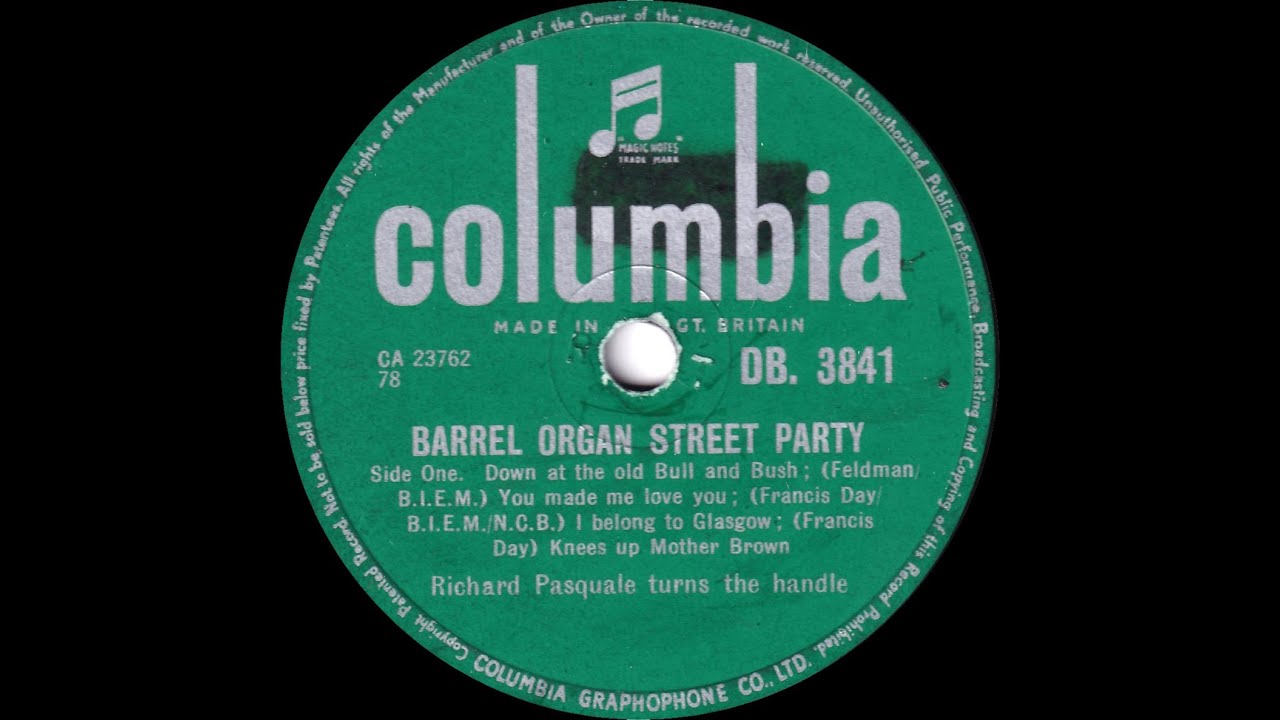This close-up photograph captures a green vinyl record label set against a black background. Prominently displayed at the top is the word "Columbia" in lowercase, with the "L" and the top of the "B" stretched tall; a musical note symbol is nestled between these letters. Below this, the text reads "Magic Notes Trademark" and "Made in Great Britain." To the left side of the label, the catalog number "CA-2376278" is noted, while to the right is "DB-3841." Encircling the rim of the label, smaller text lists song titles in paragraph form. The title of the record is "Barrel Organ Street Party." On Side One, the songs include "Down at the Old Bull and Bush," "You Made Me Love You," "I Belong to Glasgow," and "Knees Up Mother Brown." The label also mentions “Richard Pasquale turns the handle.” In the center of the label is a hole typical for vinyl records.